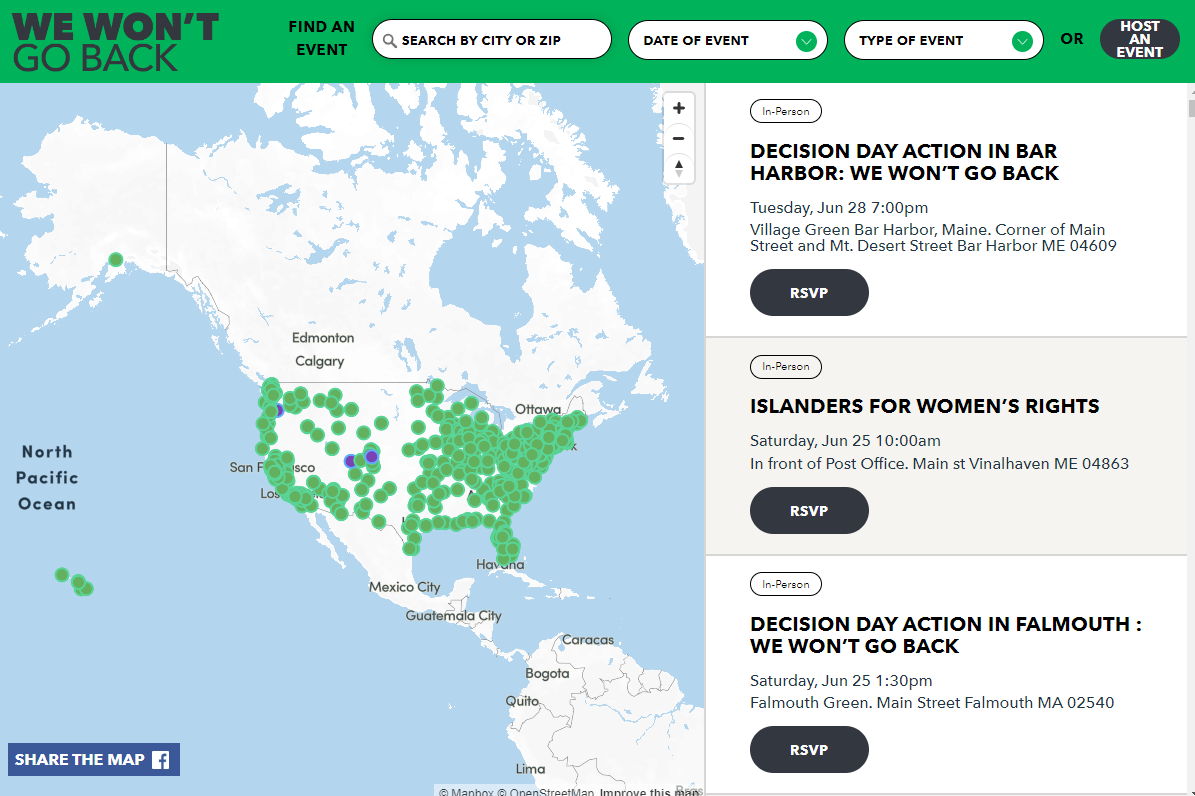The website's interface prominently features a comprehensive map on the lower-left portion of the screen, which occupies the majority of the webpage. This map displays detailed geographical information, including the entire continental United States, Hawaii, Alaska, as well as extensive parts of Canada and Latin America.

At the top of the webpage, there is a green navigation bar that includes various functions. Among them, the "We Won't Go Back" link is featured prominently. Below this are several interactive search options: a box to search by city or zip code, a dropdown menu to select the state of the event, and another dropdown menu to choose the type of event. Additionally, there is a "Host an Event" button for users who wish to organize their own events.

On the right-hand side of the screen, there is a vertically scrollable list of upcoming events, each organized in distinct rows. Examples of listed events include:

- **Decision Day Action in Bar Harbor: We Won't Go Back**
  * **Date:** Tuesday, June 28th, 7:00 PM
  * **Location:** Detailed location information provided
  * **RSVP Button:** Available below the event details

- **Islanders for Women's Rights**
  * **Date:** Saturday, June 25th, 10:00 AM
  * **Location:** Detailed location information provided
  * **RSVP Button:** Available below the event details

- **Decision Day Action in Falmouth: We Won't Go Back**
  * **Date:** Saturday, June 25th, 1:30 PM
  * **Location:** Detailed location information provided
  * **RSVP Button:** Available below the event details

Each event listing includes the title, date, time, location, and a convenient RSVP button for users to confirm their attendance.